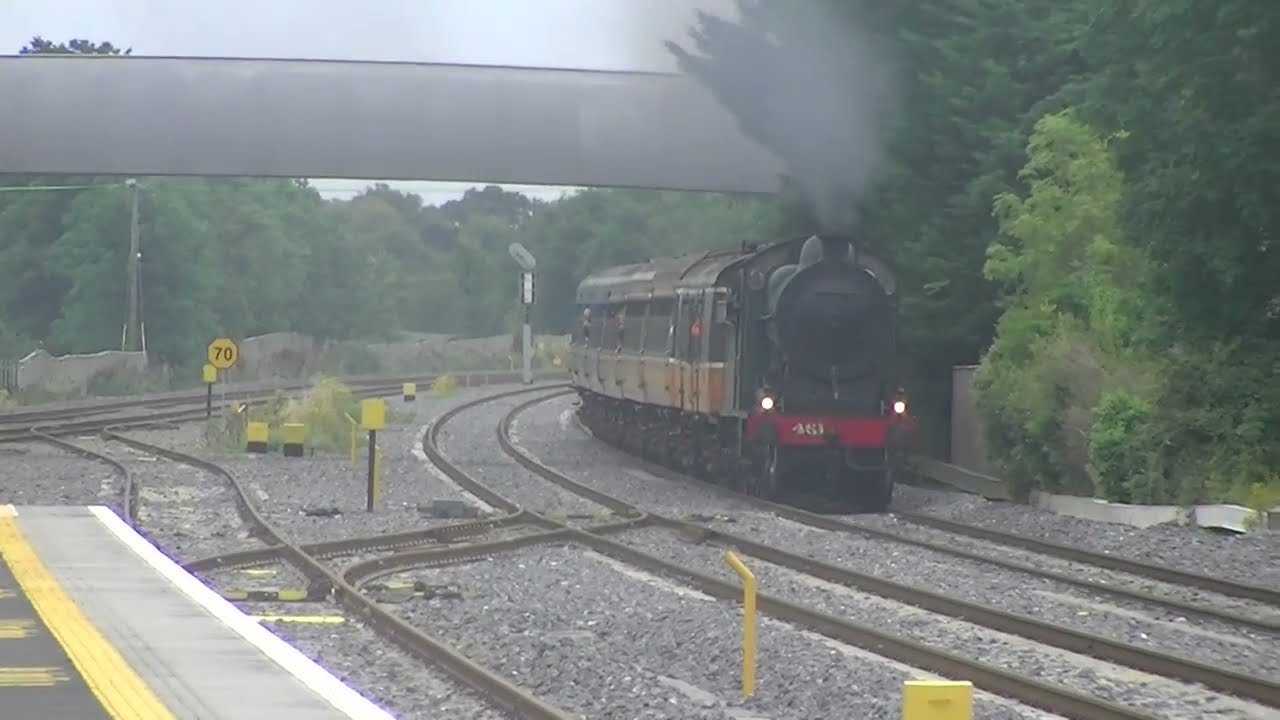The image depicts a steam engine train, predominantly black with a red stripe and numbered 461, navigating a gentle curve towards the viewer. The front of the train emits billowing black smoke from its smokestack, and it is followed by a few passenger cars painted a brownish-green color. The scene is set on a misty day, with multiple railroad tracks visible, creating a complex network beneath the train. To the left of the train is a platform, from where the photo appears to be taken. Additional tracks are situated to the right and further left in the background. Flanking the tracks, lush green trees line both sides, with larger trees and some concrete fencing seen beyond the initial foliage. The train has just passed under a modern, silver pedestrian bridge, and there is a long concrete bridge visible in the backdrop. The clarity and detail of the image suggest a high-definition capture, possibly resembling a realistic animation.